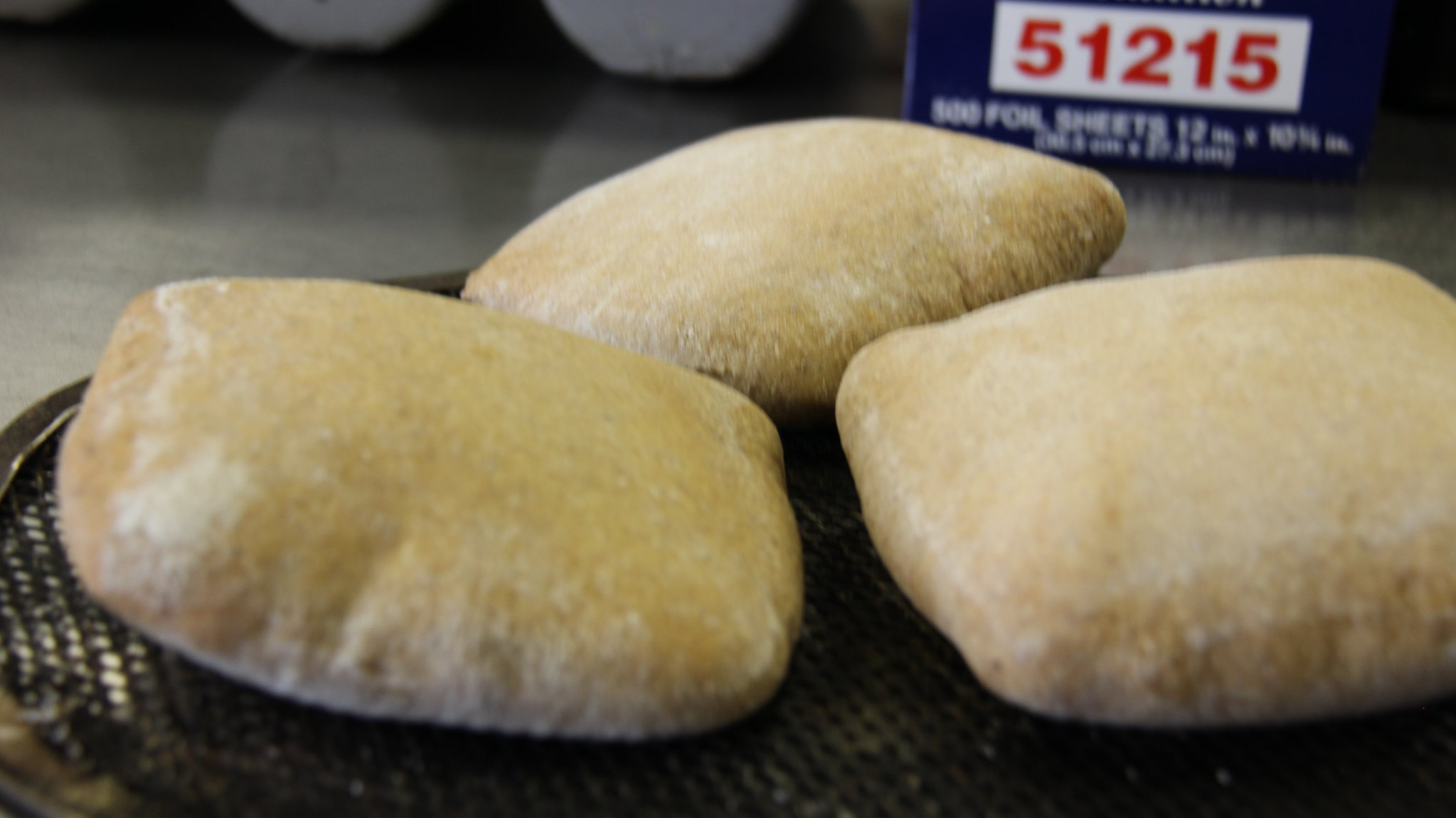The image features a close-up of three large, rectangular yeast rolls, lightly toasted to a tan or light brown color with traces of flour dusted on them. The rolls are arranged on a black plate that appears to be mesh-like or perforated, sitting atop a similar black mesh surface. Two rolls are positioned in the front and one is in the back, nearly covering the entire plate. In the blurred background, a white rectangular sign displays the numbers "51215" in red, with partially legible text below that possibly reads "foil sheets." The overall color scheme of the image includes neutral tones with a significant portion of black and gray.